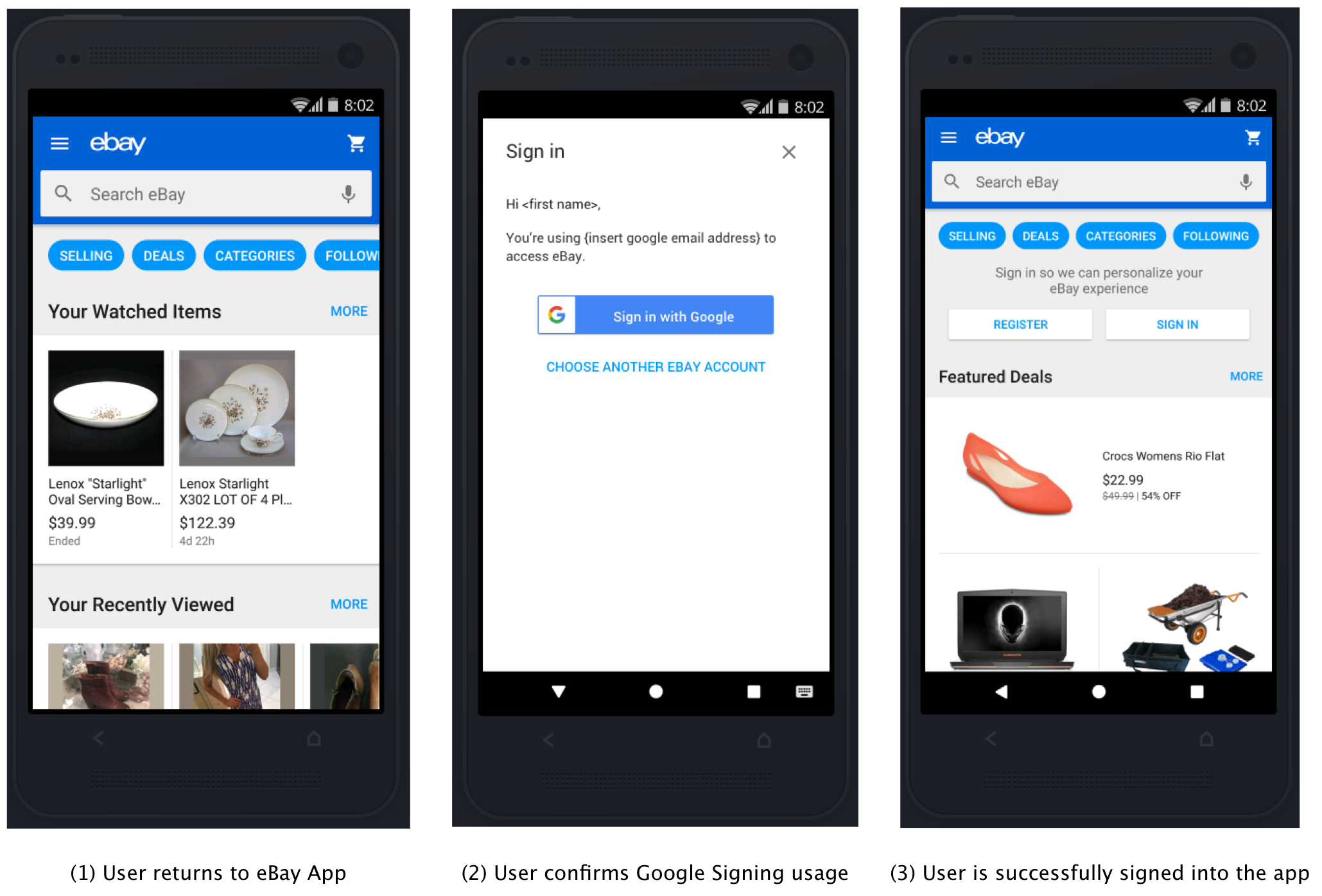This detailed triptych of screenshots presents a user's interaction journey within the eBay mobile application, displayed against a white background. The sequence, accompanied by illustrative phone bezels and labeled beneath in black text, progresses from left to right with the following stages:

1. **Screenshot 1: User Returns to eBay App**
   - The eBay app's interface showcases a blue header with white text indicating "eBay."
   - Below the header is a search bar featuring a grey magnifying glass icon on the left, placeholder text "search eBay" in the center, and a grey microphone icon on the right.
   - A light grey secondary header displays tags with white text on blue backgrounds labeled as "selling," "deals," "categories," and "follow."
   - In black bold text, the section titled "your watched items" is shown, with a blue "more" link on its right.
   - The foremost content area on a white background displays two items:
     - **First Item:** A black-backgrounded image showcasing a white dish labeled "Lennox Starlight, Oval Serving Bow..." priced at $39.99, with the status "ended" in light grey text underneath.
     - **Second Item:** A grey-backgrounded image featuring a set of white dishes with designs, labeled "Lennox Starlight, X302, Lot of 4..." priced at $122.39, with the timing "four days, 22 hours" in light grey text beneath it.

2. **Screenshot 2: User Confirms Google Signing Usage**
   - The second screenshot aligns with confirming the usage of Google sign-in. The pertinent content and visual instructions guide the user through this authentication step.

3. **Screenshot 3: User Successfully Signed into the App**
   - The third screenshot illustrates the successful completion of the sign-in process, showcasing a signed-in state of the app, confirming the user’s access and navigation within their account.

Each step is meticulously arranged to reflect the ease of access and seamless user authentication experience within the eBay mobile application.